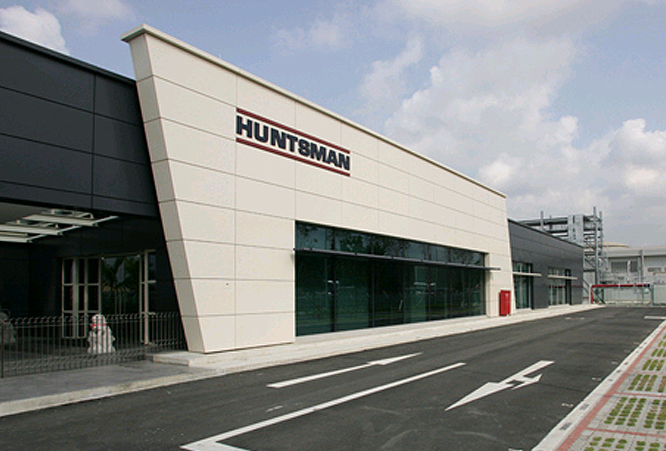The image captures the front exterior of a modern, two-story facility labeled "Huntsman" in black lettering, flanked by two brownish lines above and below it. The building, predominantly beige with black accents, has an expansive glass front showcasing its sleek design. Situated in front of the building is a black, two-lane road with directional arrows, facilitating entry and exit from the parking lot. To the left, a metal gate stands adjacent to a small plastic snowman decoration. The building's entrance is composed of large, stamped concrete with eight doors positioned to the right of a red trash can. The sky above is slightly overcast with a mix of blue and some clouds, lending a subdued light to the medium-quality photograph, which is framed to capture the entire length of the structure. No people or vehicles are present, enhancing the building's prominent and undisturbed appearance.